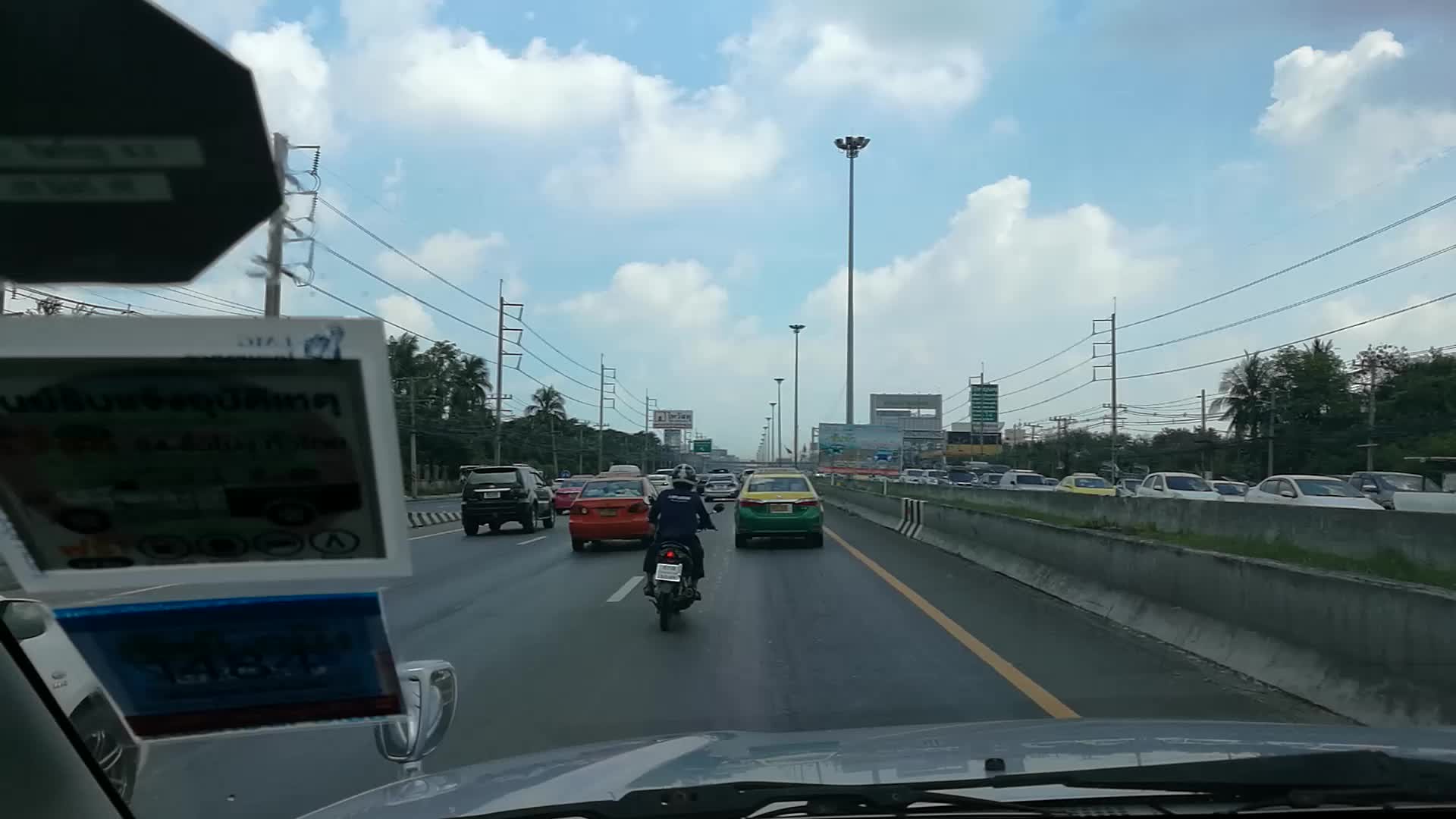This photograph appears to be taken from inside a car, either from the driver's seat or the front passenger side, providing a view through the windshield. At the bottom of the image, part of the car's hood and dashboard are visible, along with some decals and stickers on the left side of the windshield. The scene captures a busy highway with two distinct directions of traffic separated by a concrete median. In the foreground, there is a mix of vehicles, including a motorcycle and a green and yellow car. Oncoming traffic is visible, densely packed with a variety of vehicles. Large power lines and street lamps run along both sides and the center of the highway. It's a bright, cloudy day, with a blue sky dotted with white clouds. In the distance, trees, billboards, and a building can be seen, although no text on the signs is legible. The image gives an impression of gridlock, emphasizing the congestion typical of a busy highway.